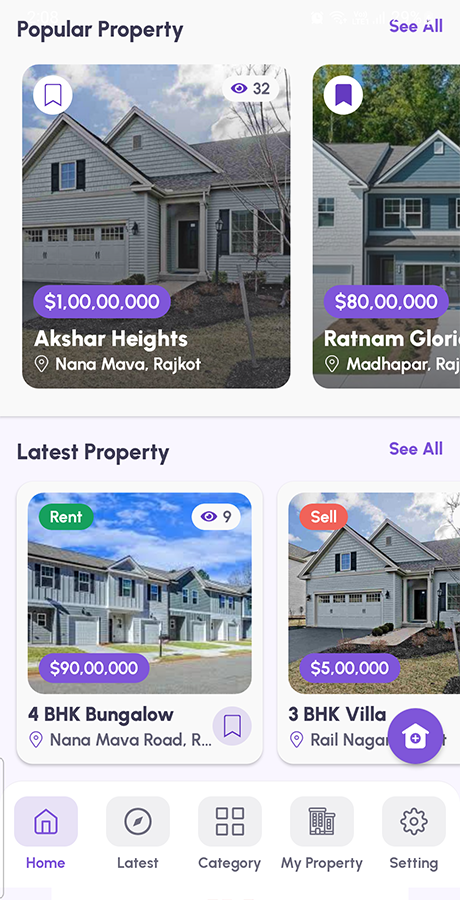This image is a cropped screenshot from a mobile real estate application, focusing on key sections of the user interface. At the bottom of the screen, there are five navigation icons labeled Home, Latest, Category, My Property, and Settings. The Home section is currently selected.

The upper portion of the image displays two sections: "Popular Properties" and "Latest Properties." Each section showcases two property listings, each with detailed information. The "Popular Properties" section features images of the properties, along with their prices, locations, and the number of views indicated by a small eye icon. Additionally, there's a bookmark icon allowing users to save these properties as favorites.

The "Latest Properties" section similarly displays two property images. Each listing provides basic information but distinguishes between properties available for rent or sale with distinct icons. This well-organized interface aids users in quickly browsing and identifying real estate options based on their preferences.